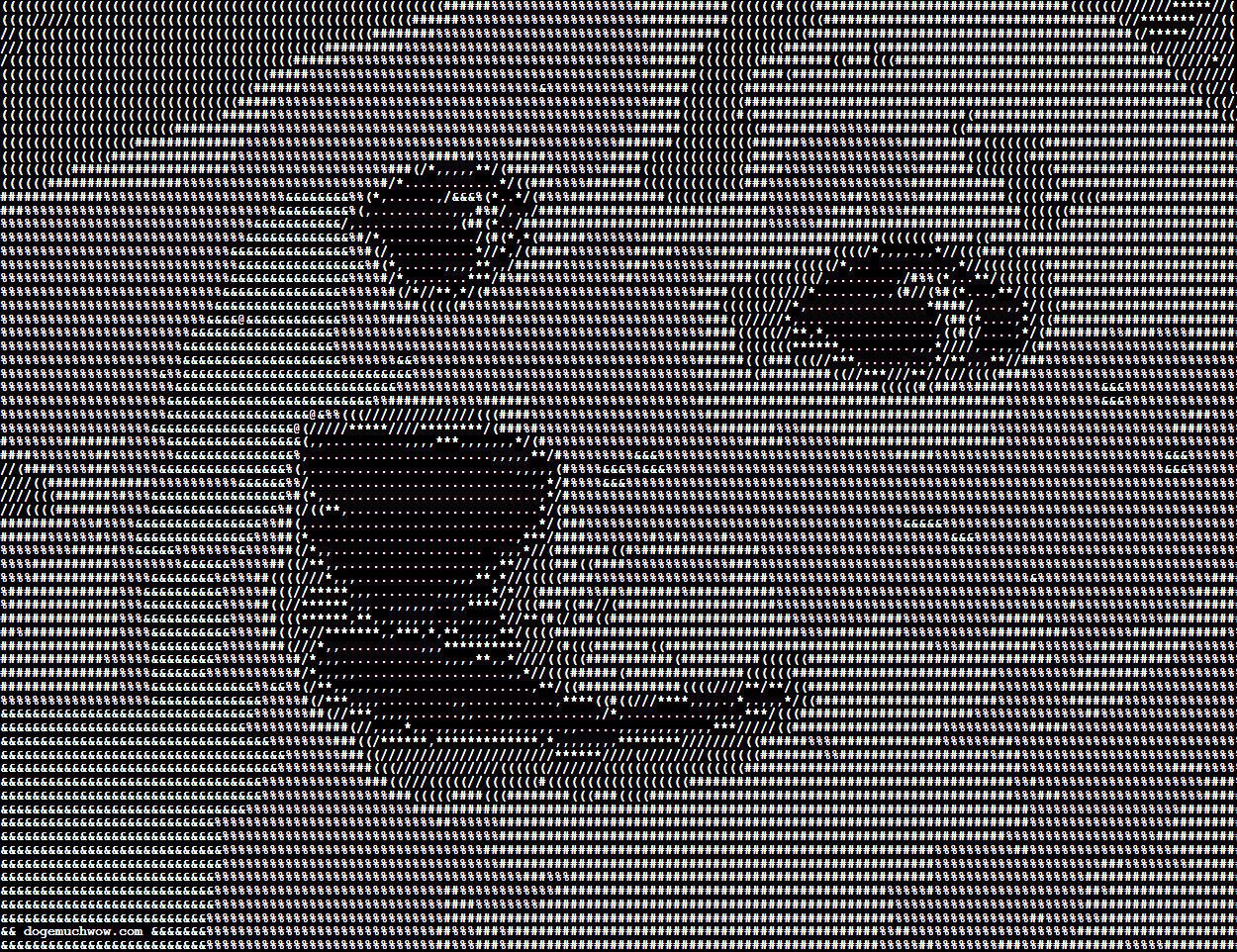The image is a pixelated rendition of a dog created using black, white, and various shades of gray dots. The composition has a grayscale background, with black dots forming distinct features like the nose, eyes, and parts of the mouth. The dog's face is discernible, although the detail isn't sufficiently sharp to determine its breed. The head and snout are visible, with an ear noticeable on the left side. There are occasional hints of purple and even minute traces of blue and red amidst the primarily grayscale palette, giving it a slightly surreal appearance. The overall effect resembles an artistic installation, akin to those pin impression toys where pins form an image based on applied pressure. The high contrast between the black and white elements emphasizes the dog's features against the gray fur, providing a unique and detailed visual.